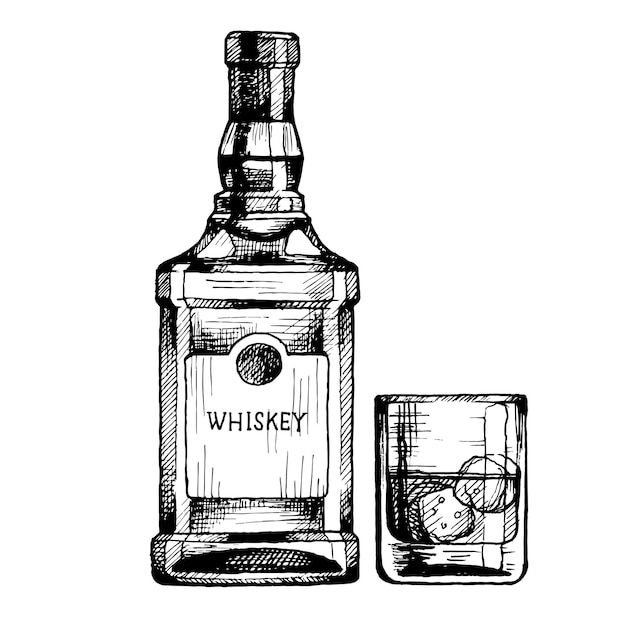This detailed sketch, rendered in black ink on a pristine white background and framed by a border, depicts a tall, rectangular whiskey bottle and a short glass beside it. The whiskey bottle, topped with a black cap, features a simple label with a black circle at the top and the word "whiskey" emblazoned beneath it. The glass, which is roughly half the height of the bottle's rectangular body, is half full of whiskey and contains two round ice cubes. One of the ice cubes is fully submerged while the other floats partially above the liquid. The artwork, characterized by extensive cross-hatching and a sophisticated line drawing technique, radiates a professional feel despite its lack of ornate details, signatures, or dates.